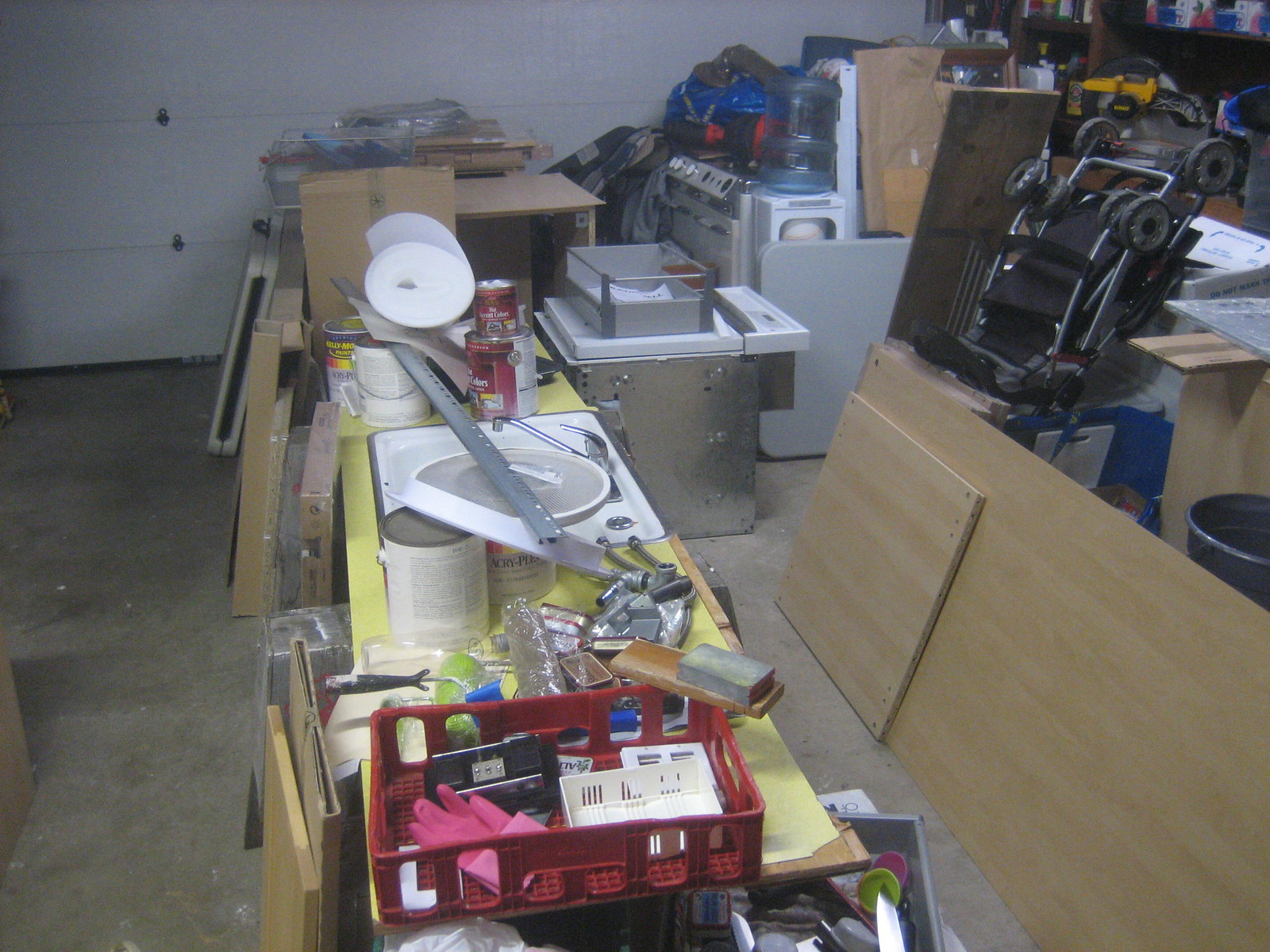The image depicts a cluttered garage, showcasing a variety of items and fixtures. Dominating the background is a white garage door, characterized by horizontal and vertical lines that create a quintessential garage door appearance. Silver hooks or tabs accentuate these lines, adding a functional touch to the structure. 

In the background, several brown shelves are laden with an assortment of items, including a Brita water jug, multiple boxes, and what appears to be an old oven. To the center and left, there are folding tables; one is unfolded and set up, covered with yellow butcher paper and scattered with tools and paint cans, while the other is folded away. Propped against the wall are long wooden panels and smaller, square-cut boards.

Additional items include a collapsed stroller and a trash can. The garage floor is a basic, hard concrete surface, typical of such spaces, and is cluttered with various objects. Notably, a red basket sits at the end of one folding table, containing pink gloves, a black item, a small white basket, and other white objects. In the background, a roll of paper towels is visible, adding to the array of collected miscellaneous items scattered throughout the garage.